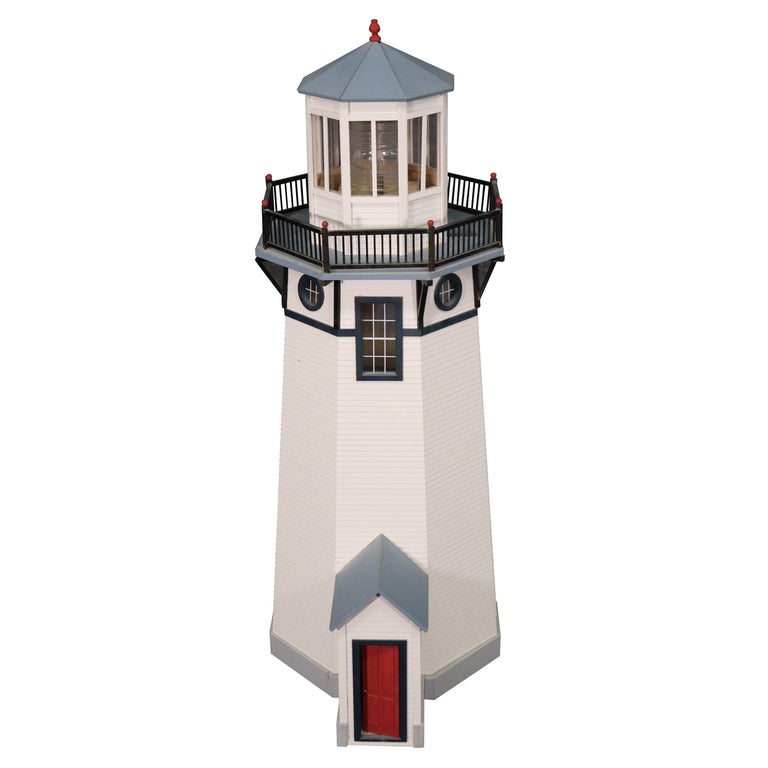This image depicts a detailed model of a hexagonal lighthouse set against a pure white background, typical of product photography. The lighthouse, seemingly crafted from wood, features a white facade with a sleek slate blue roof that culminates in a red tip at the peak. The upper section of the lighthouse houses a black railed balcony with enclosed glass panels, suggesting the presence of a functional light. Below this light enclosure, there is a rectangular window flanked by two smaller circular windows.

The structure includes an extended entryway at its base, marked by a red door with a black border and a triangular slate blue roof above it. The lighthouse rests on a grey-bordered base, adding to its stability and aesthetic appeal.

Intricate details, such as the visible lines in the wood slats, enhance the model's realism, making it suitable as a decorative piece for various settings like a garden or household interior. The photograph captures three out of the six windows, emphasizing the lighthouse's meticulous craftsmanship and its potential as a charming craft project.